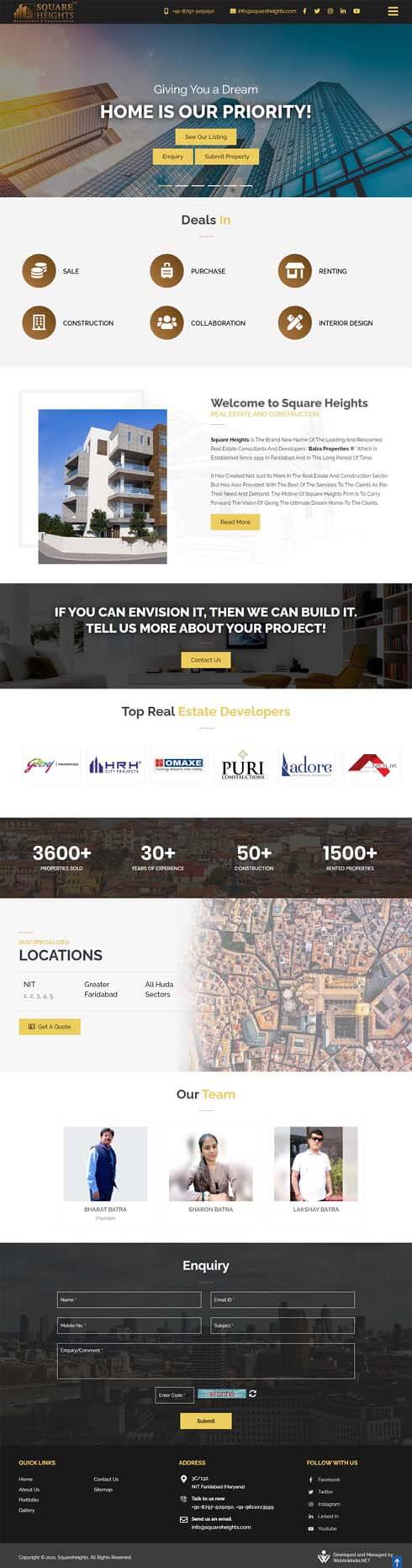**Square Heights Real Estate Developers: Your Vision, Our Priority**

Our website welcomes you with the bold statement, "Home is our priority," prominently displayed in large, white letters. This message is set against an inspiring backdrop of city skyscrapers, conveying our focus on urban development and modern living.

Below this intro, we outline our comprehensive range of services: sales, construction, purchase, collaboration, renting, and interior design. These offerings are listed clearly to reflect our commitment to meeting all your real estate needs.

We then introduce you to Square Heights with a captivating image of a residential building, emblematic of the quality and care we put into our projects. Our philosophy, "If you can envision it then we can build it," encourages you to share your project ideas with us. This statement stands out in white letters on a sleek black background, alongside a prominent yellow "Contact Us" button for easy reach.

Further down, we highlight our standing as top real estate developers, showcasing logos of our esteemed partners. Key achievements include selling 3,600+ properties, three decades of trusted service, and an impressive portfolio of over 1,500 properties across various locations.

Our dedicated team is introduced with a professional photo featuring two men and one woman, symbolizing the expertise and diversity driving our success.

Finally, we provide a user-friendly inquiry section, featuring a black background with white text boxes. Here, you'll find multiple contact options, including our hours, email, phone number, and social media links, ensuring you're always connected with us.

Welcome to Square Heights—where your dream home becomes our mission.